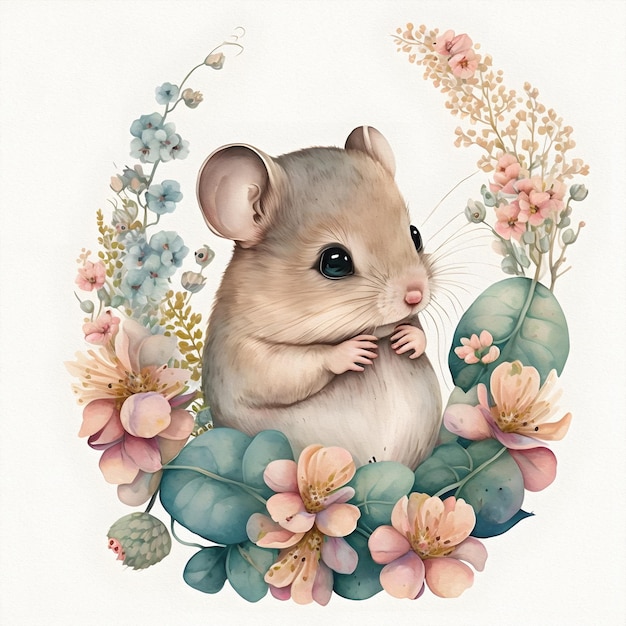This detailed illustration features an adorable, chubby little mouse depicted with a coat of soft tan fur and lighter beige on its belly. The mouse, facing to the right, is sitting upright with its round ears perked up, and its little paws held close to its cute pink button nose and whiskers. Its bright, shiny black eyes give it a lively, endearing look. This charming scene is set within a semi-circular arrangement of flowers and foliage, resembling a partial wreath. To the left, clusters of light blue flowers fade into pink blossoms, complemented by eucalyptus green leaves. On the right side, pink flowers in various stages of bloom mingle with gold-tinged petals. The entire composition is rendered in a muted pastel color palette, creating a soft, dreamy aesthetic. This clip art or PNG image, potentially ideal for crafting or greeting cards, is both whimsical and visually appealing.